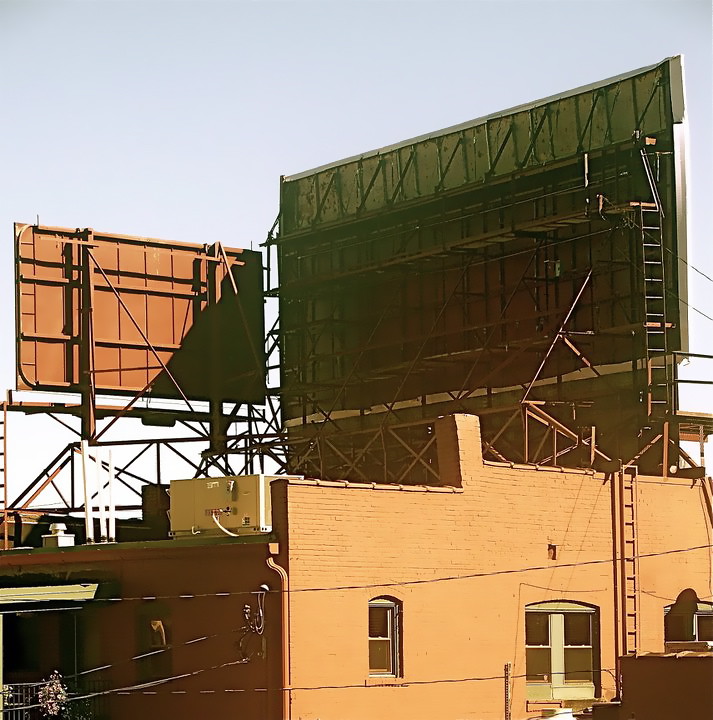The photograph captures a vintage, somewhat faded scene of an old, light orange-brick building with a flat roof and aged windows. On the left-hand side of the structure, partly visible behind the building, is the back of a smaller rectangular dark brown billboard. On the right-hand side, a much larger square green billboard stands, supported by several metal pipes that extend diagonally. A ladder leans against this larger billboard, allowing workers access for maintenance or construction. Additionally, there is another ladder fixed to the wall of the building itself, leading up to the rooftop where a generator or air conditioning unit can be seen. Power lines stretch across the image in front of the building, adding to the historic feel. The sky above is a clear, bright blue, without any clouds, enhancing the clarity of this daytime scene.